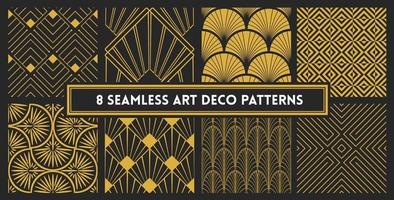The image features a montage composed of eight distinct vignettes, each showcasing a unique seamless Art Deco pattern, prominently labeled with the text "8 Seamless Art Deco Patterns" in white font. The vignettes are arranged in a grid of four on the top and four on the bottom, each bordered in black for clear separation. The patterns exhibit geometric designs typical of the Art Deco era, including motifs like scallops, diamonds, leaf-like shapes, and squares. The overall color scheme is predominantly a gold and black palette, reminiscent of the lavish, elegant style associated with the 1920s, akin to the Great Gatsby aesthetic. While all patterns share the gold-black theme, they vary in density and boldness, with some featuring more intricate gold designs and others presenting more black background for contrast. The image, though slightly blurred, captures the essence of Art Deco's opulence and geometric precision.